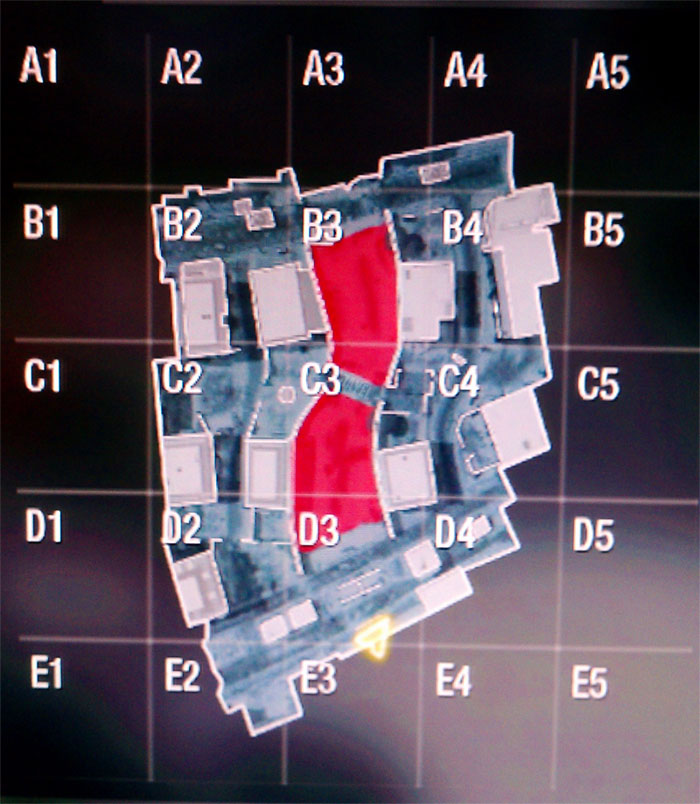The image depicts a dark background overlaid with a five-by-five grid of squares, each delineated by thin white lines and labeled with white uppercase alphanumeric coordinates. The top row reads A1 through A5, followed by subsequent rows B1 through B5, C1 through C5, D1 through D5, and E1 through E5.

In the center of the grid is a roughly rectangular formation outlined in white, resembling a map or board game arrangement. This formation extends from B2 to B4, spans down to E2, and reaches the right border at D4, giving it an angled, diagonal appearance. Inside this shape, there is a prominent red rectangular object occupying B3, C3, and partly D3, suggestive of a central marker or key feature.

Surrounding this central red object are various white rectangular shapes scattered across the grid, reminiscent of pieces from a battleship game. These elements are interspersed within the outlined formation, contributing to the map-like structure.